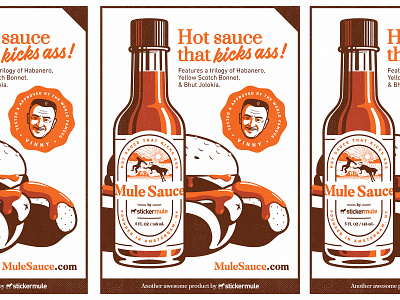This image appears to be a vibrant, cartoon-style advertisement for a hot sauce, likely called "Mule Sauce." The focal point is a stylized bottle of hot sauce, which has a brownish-red hue and a glossy shine. The label on the bottle features the text "Mule Sauce" and a small illustration of a mule kicking a person. Positioned in the middle top is bold orange text in a mix of cursive and standard fonts that reads "Hot Sauce That Kicks Ass." Below this, black text details that the sauce features a trio of flavors: habanero, yellow Scotch Bonnet, and another variety. On the right side of the image, there's an orange sticker with a man’s face and white text. In the bottom right corner, the URL "mulesauce.com" is clearly visible. The background depicts a cheeseburger and a hot dog, each with hot sauce dripping off them, reinforcing the product’s application. The entire composition is presented with a brownish-orange tint on a white backdrop, creating a cohesive and eye-catching design.